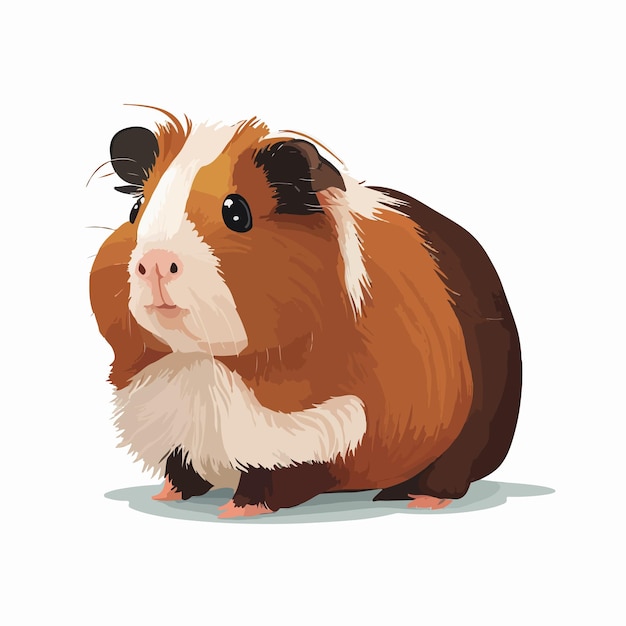This cartoon-style drawing depicts a charming guinea pig positioned in an indoor setting. The guinea pig features a distinctive color pattern: a black rump, a white middle body, a brown head with a white stripe running from its forehead to its mouth, which is pink. It sports big black eyes, black front paws, and peachy-pink hind paws. The creature's ears are dark brown with tufts of white fur. The pink nose contrasts with its textured fur, drawn to show subtle lines and shading. The guinea pig, poised at a three-quarter angle, appears to be looking slightly off to the side, giving it a serene, adorable expression. A shadow beneath adds depth to the animated image, emphasizing the 3D rendering. The image is text-free, focusing solely on the detailed and lifelike portrayal of the guinea pig.